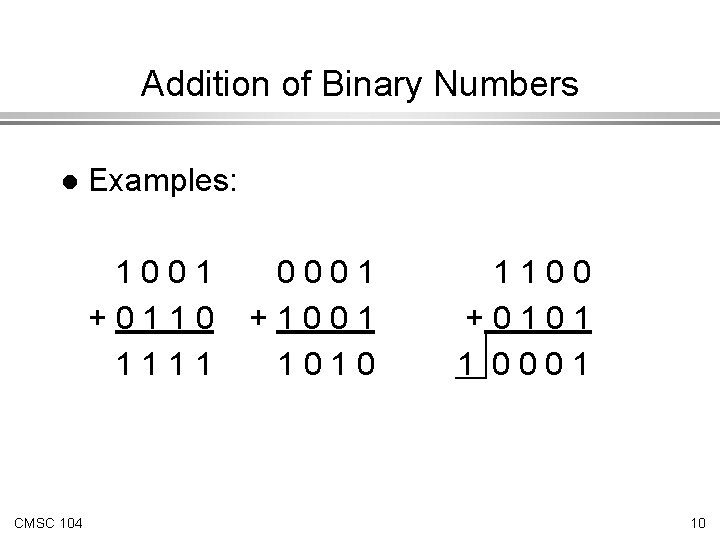The image features an instructional schematic, likely from a math textbook or a child's worksheet, demonstrating the addition of binary numbers. Set against a white background, the phrase "Addition of Binary Numbers" is prominently displayed at the top in a simple black, sans-serif font. Below this, two gray stripes, one wide and light gray and the other narrow and dark gray, underline the title.

On the left side of the image, a bullet point labeled "Examples:" introduces three binary addition equations. The first equation is 1001 plus 0110, displayed vertically with the sum 1111 beneath a horizontal line. The second equation, 0001 plus 1001, similarly shows a vertical arrangement with the result 1010. The third equation differs slightly, showing 1100 plus 0101 with the sum depicted as 0001, but also including a vertical and horizontal line with a 1 in it, indicating a carry-over to form 10001.

In the bottom corners, additional text reads "CMSC 104" in the bottom left, which might denote a course number, and "10" in the bottom right, likely indicating the page number. Overall, this plain, black-text-on-white schematic serves as a clear, concise guide to understanding binary addition.